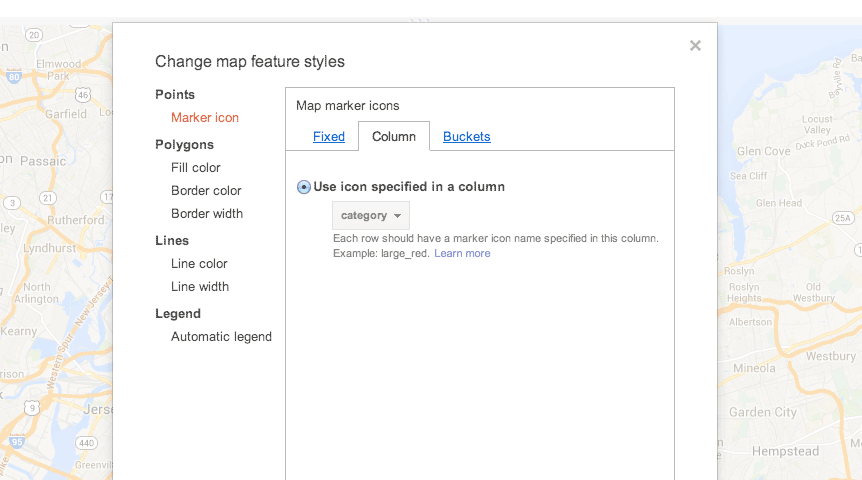The image is a detailed screenshot displayed in landscape mode, likely taken from a tablet, laptop, or smartphone. The background of the image is a classic road map of a region in the United States, specifically focusing on parts of New Jersey. On the left side of the map, towns such as Passaic, Rutherford, Lynnhurst, and Kearney are clearly labeled, while the right side features towns like Old Westbury, Westbury, Garden City, Hempstead, and Glen Cove.

The roads on the map are highlighted in yellow, accompanied by interstate icons and U.S. highway shield-shaped icons, providing a typical road map layout. Superimposed on this map is a prominent white dialog box with an "X" in the top right corner, allowing users to close the box and return to the map.

The dialog box offers a variety of customization options for the map under the heading "Change Map Style Features," with sections for "Points," "Polygons," "Lines," and "Legend." Currently, the "Points" section is active, as indicated by the highlighted "Marker Icon in Red." Within this section, there's another box titled "Map Marker Icons," which provides options to choose "Fixed," "Column," or "Buckets" styles. The "Column" option is selected, evidenced by its tab-like shape and the active blue radio button.

This option is set to "Use Icon Specified in a Column" and includes a dropdown menu labeled "Category," with additional instructions below stating, "Each row should have a marker icon name specified in this column." An example given is "large_red," with a clickable "Learn More" link for further instructions.

On the left-hand column, other options under "Polygons" include "Fill Color," "Border Color," and "Border Width." The "Lines" section allows customization of "Line Color" and "Line Width." Finally, the "Legend" section offers an "Automatic Legend" option.

This image provides an intricate view of the map editing interface, showcasing various tools and options available for detailed map customization.